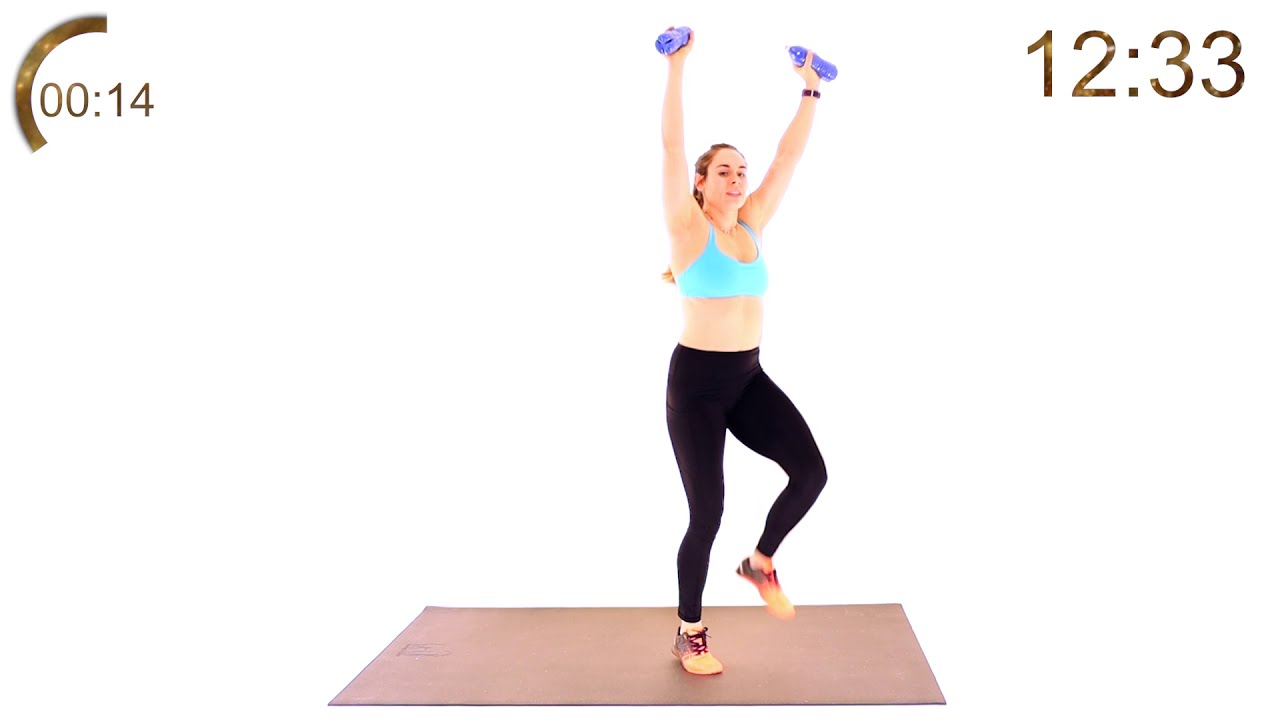The image depicts a young woman in mid-workout, standing on a yoga mat, possibly as part of a workout video or game. She is dressed in black leggings, a turquoise sports bra, and orange and black sneakers. The woman, who has a lighter skin complexion, is holding blue hand weights, one in each hand, with her arms raised above her head and one leg lifted, indicating she is in the midst of a specific exercise move. The background is solid white, enhancing the bright and clear quality of the image. In the top left corner of the image, there is a timer showing "00:14," possibly indicating the time left in this exercise segment. In the top right corner, there is a timestamp reading "12:33," likely displaying the current time.